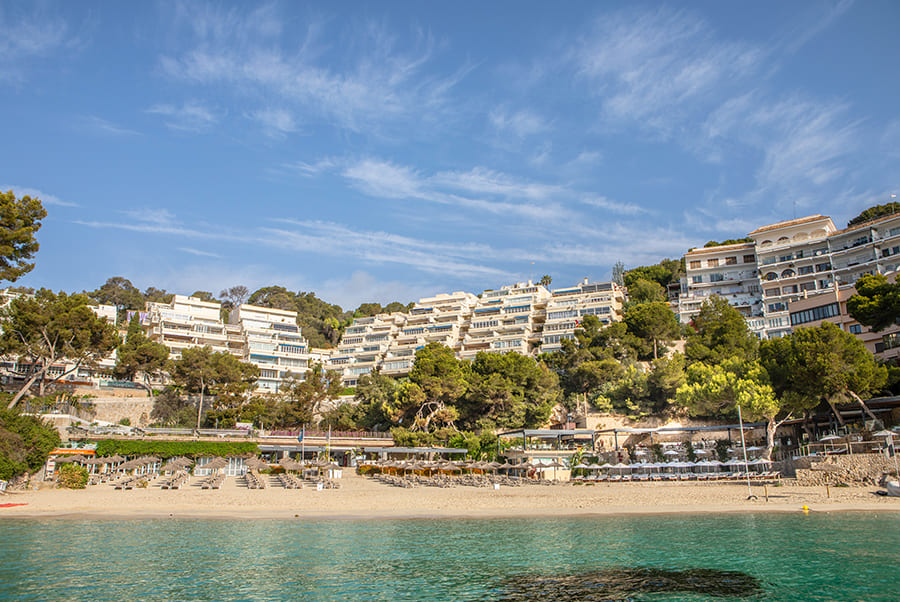The image depicts a stunning aerial view of a luxurious island resort nestled into the cliffs of a picturesque coastline. In the foreground, crystal-clear turquoise waters gently lap against a light sandy beach, where rows of orderly arranged chairs, tables, and umbrellas await guests. Scattered along the beach are small boats, resting unused. Lush greenery, including tall palm trees, separates the beach from the impressive, multi-level tan and white apartment buildings and villas that are terraced into the hillside. These structures, rising four to five stories high, feature numerous balconies and terraces designed to offer breathtaking oceanfront views. The entire scene is bathed in the bright sunlight of a clear day, under a sky filled with wispy white clouds. The natural beauty of the water's edge, possibly revealing glimpses of a reef beneath the surface, adds to the idyllic and serene ambiance of the resort.